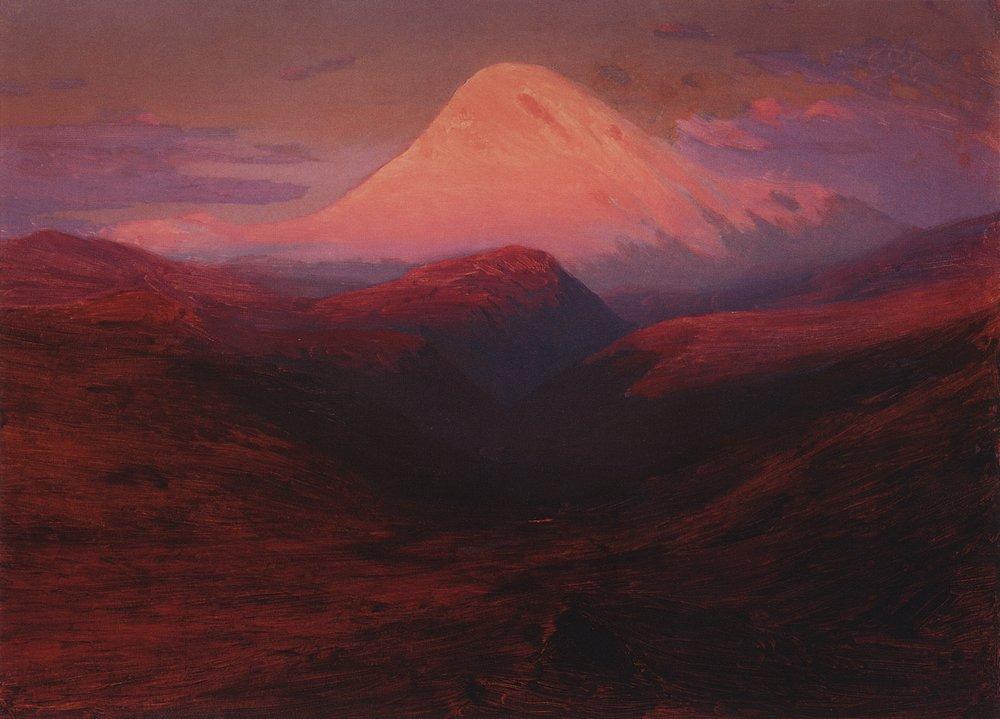The painting "Elbrus in the Evening" by Arkhip Kuindzhi, created in 1908, showcases a realistic landscape in vibrant tones. Dominating the upper section, a grand snow-covered mountain peak rises majestically, its smooth slopes curving gently to a flat, prominent face centered in the composition. The mountain's snowy expanse, almost entirely cloaked in white, contrasts sharply with the darker, brooding sky painted in hues of purples and grays.

In stark contrast, the foreground reveals a rugged, hilly terrain rendered in striking shades of red, brick, and deep browns. This barren landscape is devoid of vegetation, characterized by its rocky texture and a dark valley cutting through the center, leading downward from a prominent ridge. The entire scene, set in a landscape orientation, vividly captures the serene yet dramatic essence of an evening view of Mount Elbrus.